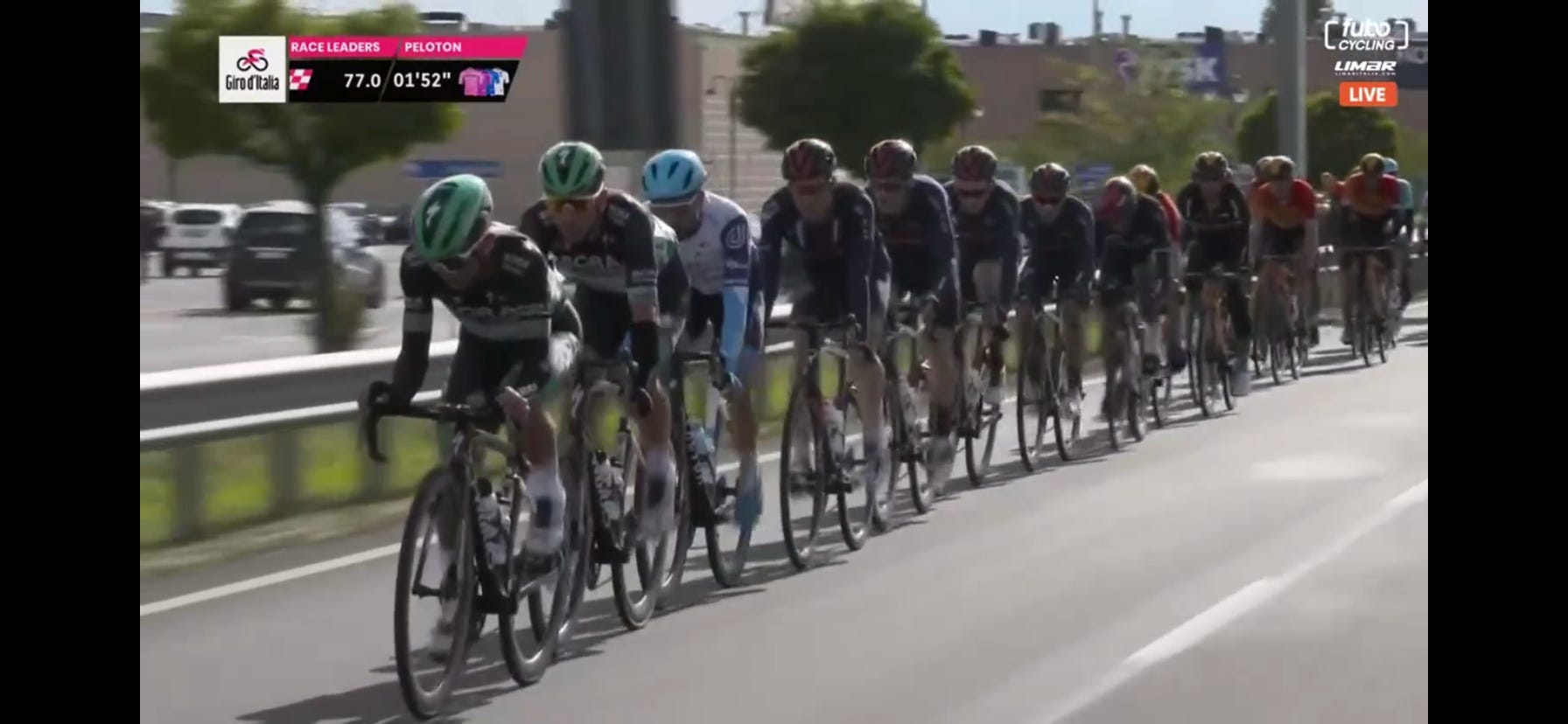The image depicts a line of cyclists engaged in what seems to be an Italian bicycle race, evident from the live TV broadcast information displayed on the screen, which reads "Fubo Cycling" and "Tubo Cycling Limar." The broadcast features a red box with the word "live" in white lettering at the top right corner. The cyclists, amounting to roughly 12 to 18 riders, are on street racing bikes with thin tires, wearing standard cycling gear including bicycle shorts and tight-fitting, long-sleeve shirts. They also have helmets, with the first two cyclists sporting matching green helmets, and the third wearing a light blue one. The image, likely taken during the early stage of the race, features the cyclists riding in a line down a city street. The background reveals a few trees, a wall, and possibly a large brown building with chimneys. At the top of the image, a mostly clear sky can be seen. On the left side of the screen, there is a graphical overlay with race information, including a small white and pink flag, numerical data showing “77.0” and “01:52”, and a mention of race leaders by name with the term "Peloton." The uniform colors present include green, black, white, light blue, pink, and brown. A white line at the lower right of the image marks the boundary of the race lane.